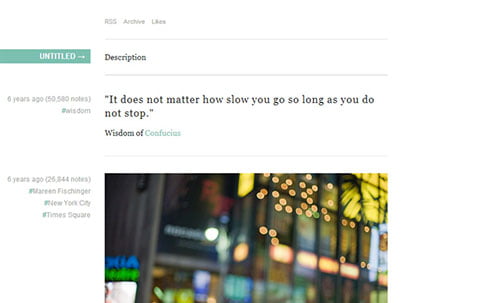This screenshot, captured in landscape mode and likely taken from a tablet or laptop, is quite blurry, making it challenging to discern intricate details. The interface appears to be displayed in portrait orientation. The background is predominantly dark, with white text and interface elements.

On the left side of the image, there are two columns. The first column begins with a green button labeled "Untitled." Below this button, the text "Six years ago" is followed by "50,580 notes." Due to the blurriness, the text beneath this is unreadable, but further down, the caption "six years ago" appears again, this time with "25,000 something notes." Hashtags like "#NewYorkCity" and "#TimesSquare" are partially visible.

The second column at the top starts with labels "RSS," "archive," and "likes," which seem to be tags or menu options. A light gray line stretches from these labels to the right side of the image. Below this, the word "description" appears in bold, with another gray line beneath it. The phrase "It does not matter how slow you go so long as you do not stop" is prominently displayed, attributed to the "Wisdom of Confucius," with "Confucius" highlighted in light blue, likely indicating a clickable link.

Dominating the bottom section of the image is a very large, blurry photograph of a city at night. The cityscape is vibrant with numerous lights, suggesting a modern, metal-structured metropolis. This visual element underscores the theme of the website, which appears to focus on inspirational quotes and urban imagery.